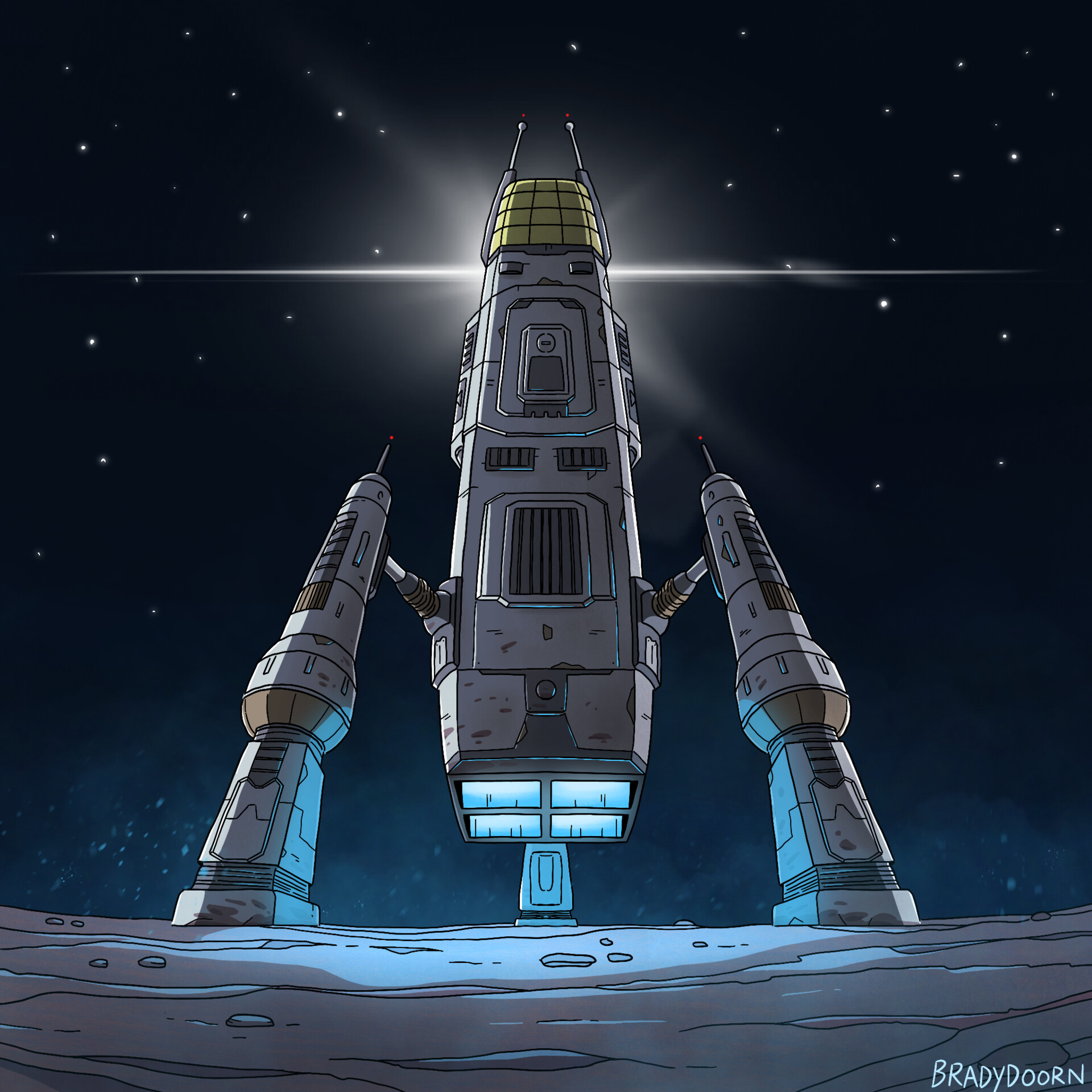This is a highly detailed comic book-style artwork depicting a large, transformer-like spaceship. The spacecraft features two leg-like structures on each side, shaped like missiles, attached to a vertically larger, pointy central body. It’s primarily gray in color, adorned with blue lights at the bottom part. The upper section includes several antennas and a gold grid. The backdrop reveals a dark, starry sky with a prominent white light reflection behind the vessel, suggesting an outer space environment, possibly on the surface of a rocky planet or moon. The ship rests on a plain, gray, rocky surface. The detailed lighting accentuates its intricate design and gives a glow to the ground below. The artist’s signature, "Brady Dorn," is visibly inscribed in the bottom right corner of the image.